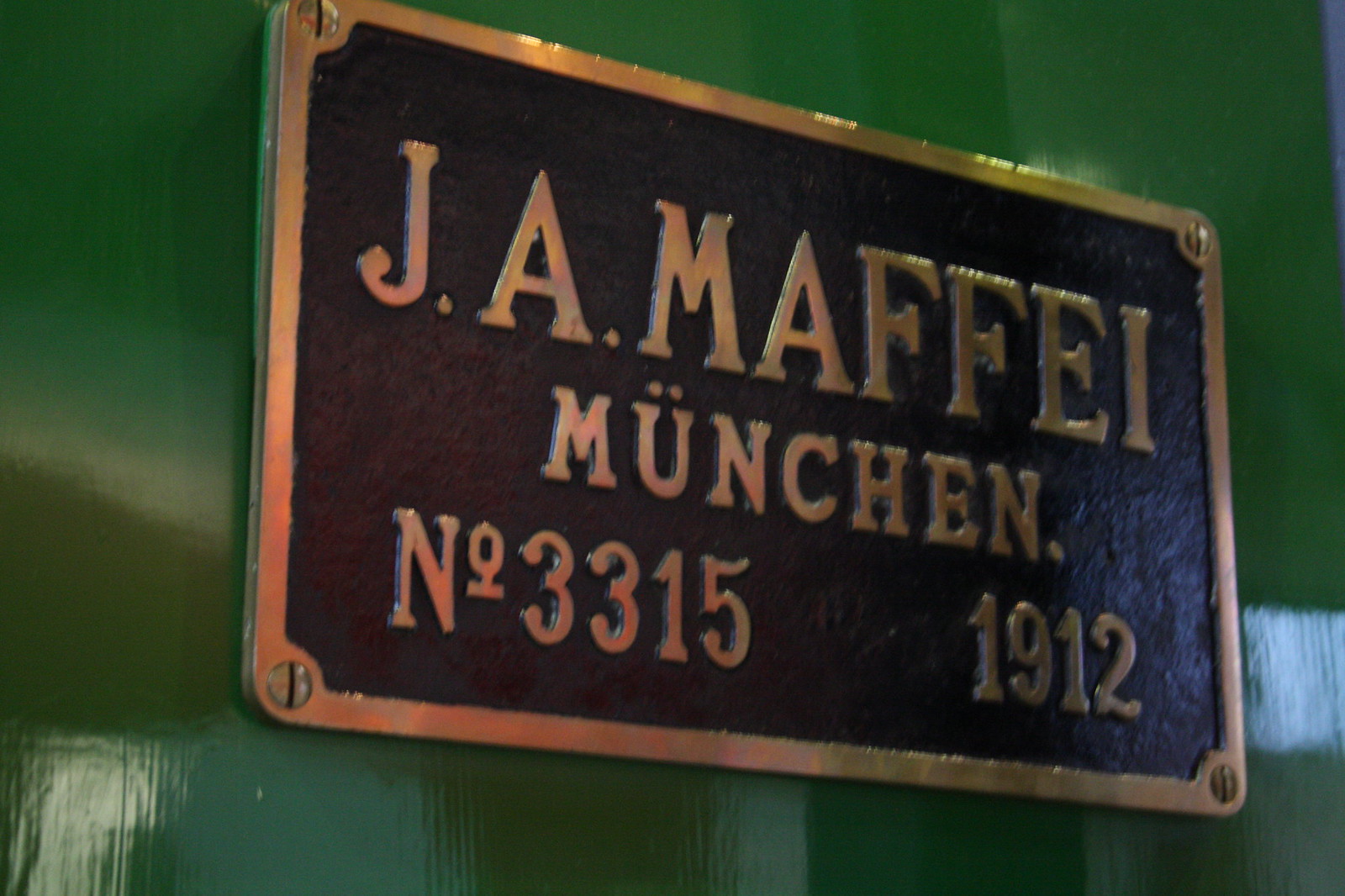The image captures a close-up of a brass nameplate with a gold border and finely engraved gold text, set against a solid brown background. The sign, which appears to be made of solid metal with a highly reflective coating, is affixed by large screws at each corner to a bright green wall. The inscription on the plaque reads "J.A. Maffay Munchen, number 3315, 1912." Light reflects off the right side and bottom left of both the wall and the sign, highlighting the gleaming surface of the metal and the vibrant color of the wall.